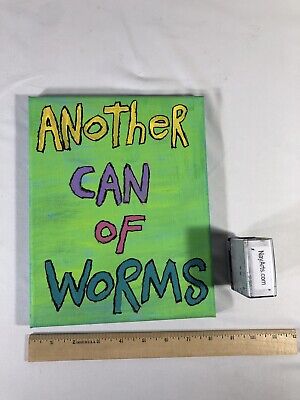The image features a vividly painted canvas that reads "Another Can of Worms." The canvas has a green background with visible horizontal brushstrokes. The phrase "Another Can of Worms" is stylized with colorful letters: "Another" in yellow, "Can" in purple, "Of" in pink, and "Worms" in a dark greenish-blue, all outlined in black. Below the canvas, a beige ruler indicates the painting measures about 8 inches in length. To the right of the canvas and ruler, there is a small grey, silvery box, possibly resembling a tape measure or stamp, with some writing on it that appears to be "somethingarts.com." Everything is arranged on a slightly wrinkled white background with shadows cast to the left, suggesting the light source comes from the right. The brightness of the painting's colors contrasts with the muted tones of the other objects, giving the image a balanced yet dynamic composition.